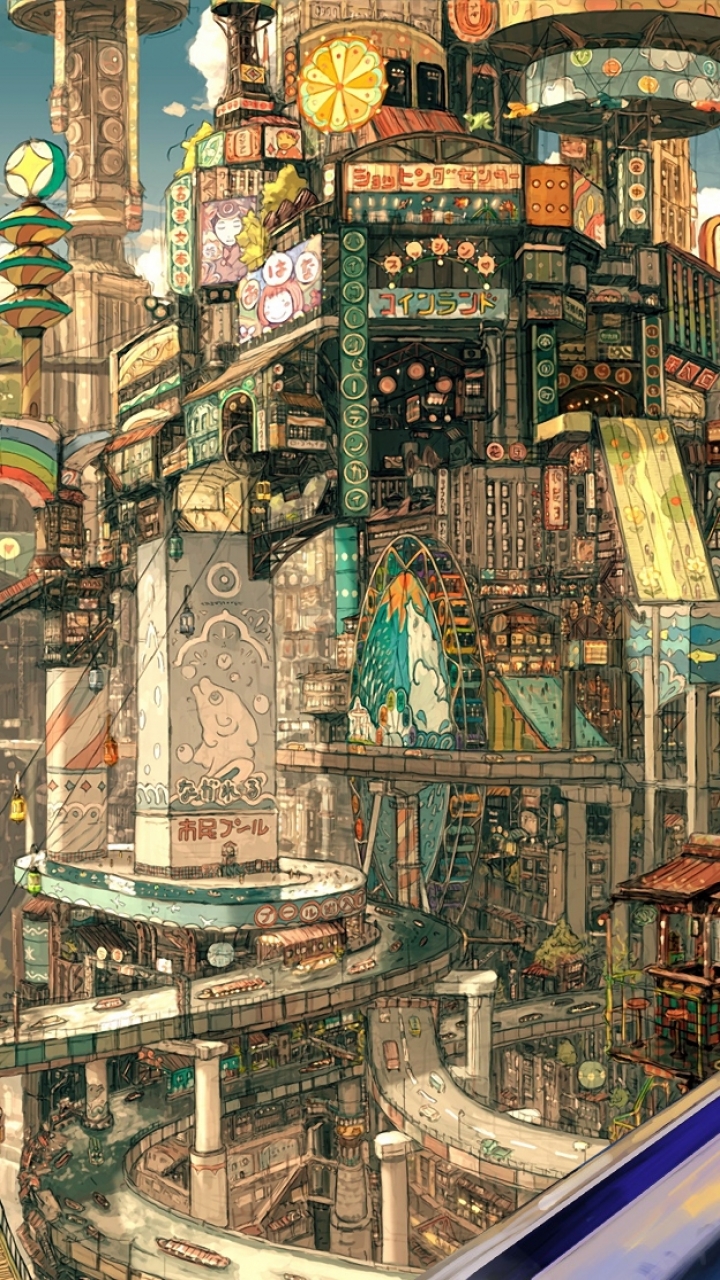This intricate rectangular art piece, approximately twice as tall as it is wide, portrays a vibrant, semi-futuristic cityscape brimming with complexity. Dominated by multicolored structures, the image presents an array of high-rise buildings stacked atop one another, resembling a towering mall that stretches into the sky. Central to the scene are tiered highways, which cascade and wind around the city like roller coasters in an amusement park. These highways, supported by large pillars, are designed with multiple levels, each tier elevating drivers higher within the urban sprawl. The roads, encased by small fences, circle around various buildings, including two notable rectangular structures. One building features a creature on its facade, while the other exhibits a striking white and red cascading stripe pattern with red, blue, and diamond-shaped accents. Amidst the architectural marvels, a prominent Ferris wheel marks the center, surrounded by clouds and other colorful elements, enhancing the fanciful and elaborate nature of the scene. The sky at the top of the image encapsulates the surreal environment, dotted with soft clouds, making the entire scene feel both fantastically utopian and densely packed with architectural wonders.